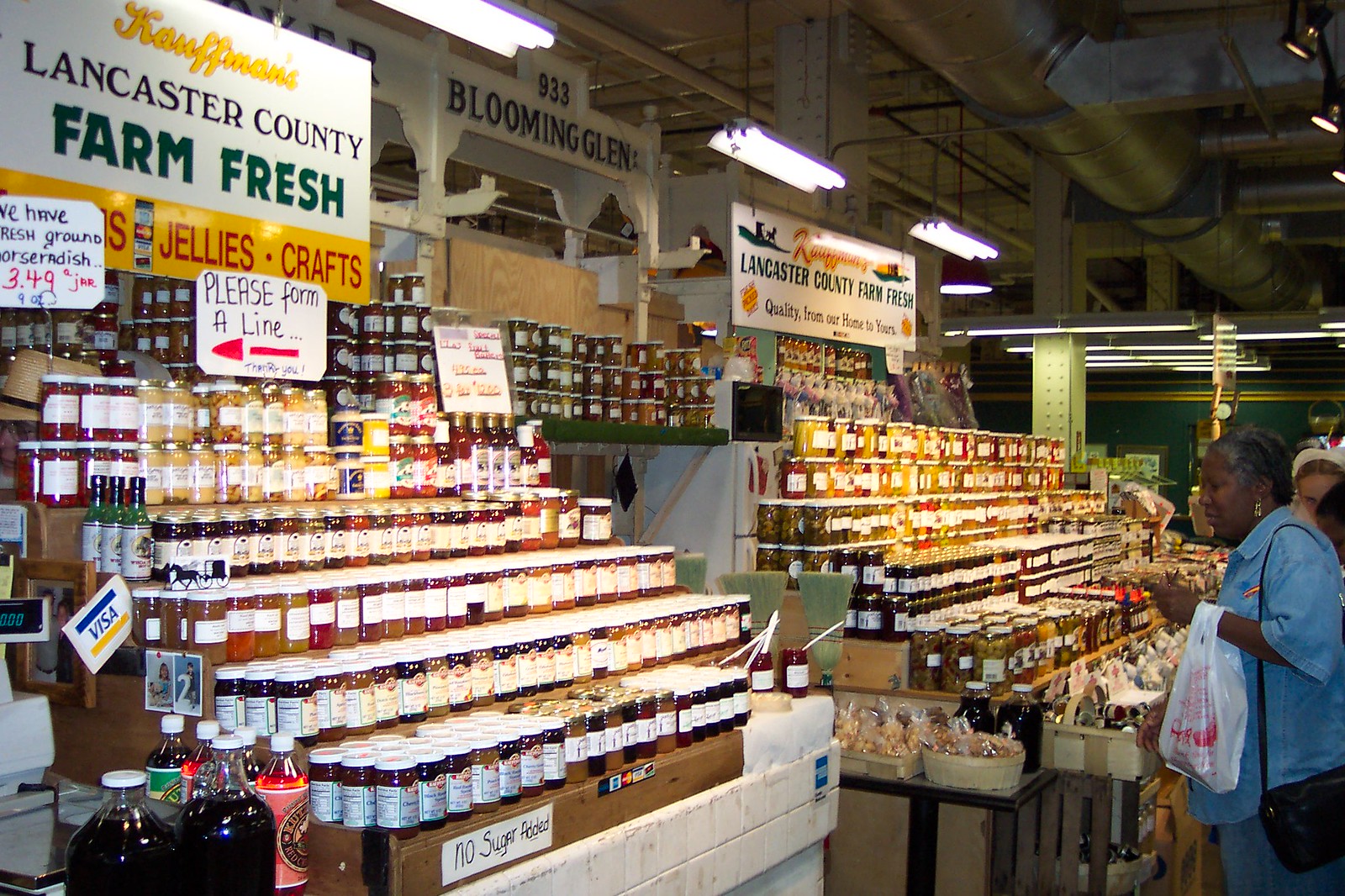Inside a bustling market, two shelves brimming with an array of mostly cylindrical bottles filled with various foods catch the eye. Prominently, a sign above the shelves reads "Lancaster County," and below that, in green capital letters, "Farm Fresh." Beneath, on the left side, there are two small yellow rectangles; the left one is partially obscured, showing only the letter 'S' as its last character. The right rectangle reads "jellies.crafts." Nearby, another white sign instructs, "Please form a line," with a red arrow pointing to the left.

On the right, a sign identical in style states "Lancaster County Farm Fresh" in one line, followed by the phrase "quality from our home to yours," without the yellow rectangles. The market scene includes a dark-skinned woman in the foreground to the right, dressed in a blue suit and holding a white plastic bag, engrossed in browsing through the numerous jars of jellies on display. The store, clearly spacious, shows a lively environment with a few other shoppers visible in the background.